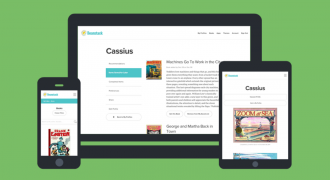In front of a green background, this image showcases three electronic devices displaying various layouts of a website. Starting from the left, there's a phone layered on top of a larger tablet, and next to them is a smaller tablet. Each device displays the website differently, highlighting its responsive design capabilities. The phone, positioned on the left, shows the website with a top menu and a comic image underneath. The menu is white with separated options, where the active one is highlighted in a bluish-green color. The larger tablet, revealed beneath the phone, presents the website with a left-hand sidebar menu and the main content on the right, accompanied by a top bar with additional options. The smaller tablet features the comic title, "Cassius," along with accompanying pictures, displaying a different layout and content focus. Although the text on the larger tablet is too small to read, it is evident that the site is designed to adapt beautifully to each screen size. The comics visible across the devices feature vivid imagery, with the one on the phone and larger tablet having a red background and characters, while the comic on the third device appears to differ from the first two.